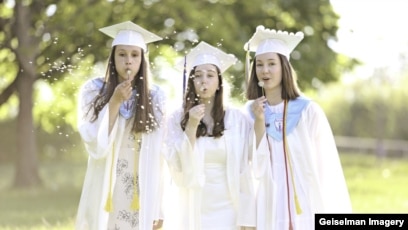The image depicts a joyful outdoor scene of three young girls celebrating their high school graduation on a sunny day. They are all dressed in traditional white graduation caps and gowns, with the two girls flanking the middle adorned with distinctive tassels—yellow around the neck of the girl on the left, and brown and yellow on the girl to the right. Each girl has brown hair, with the one on the right sporting a shorter hairstyle. They are positioned in front of a picturesque backdrop comprising a green field and lush, leafy trees, and are engaged in blowing bubbles from plastic sticks. The natural light adds to the vibrant and lively atmosphere. At the bottom right of the image is a watermark that reads "Geiselman Imagery," displayed in white font on a black border.